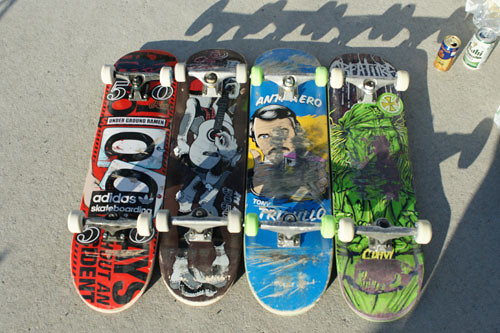This photograph captures the underside of four colorful skateboards, neatly aligned vertically from the bottom to the top. The skateboards are positioned upside down on a gray cement surface, creating shadows that suggest the photo was taken on a sunny afternoon, with the sun in the bottom left corner. From left to right, the skateboards showcase unique designs:

1. The leftmost skateboard features a red background with various numbers, including a prominent sideways "00," and some indistinct lettering, potentially reading "YS" and "confident." A sticker with "Adidas skateboard" is also visible.
  
2. The next skateboard appears in black, white, and red hues, displaying images of guitars and a man in a black tank top with a guitar strapped to his back. It has white wheels.

3. The third skateboard stands out with its blue and yellow design, featuring a man's face and the word "antihero" partly obscured by the wheels, which are green.

4. The rightmost skateboard showcases a bright green background with an image resembling the Hulk, although the design is heavily worn from use. This one also has white wheels.

In the upper right corner of the photograph, there are two opened drink cans, one blue and gold and another white and green, suggesting the presence of skaters enjoying a sunny day. The vibrant and well-loved skateboards, filled with diverse stickers and graffiti-type graphics, create a visually engaging scene against the urban backdrop.